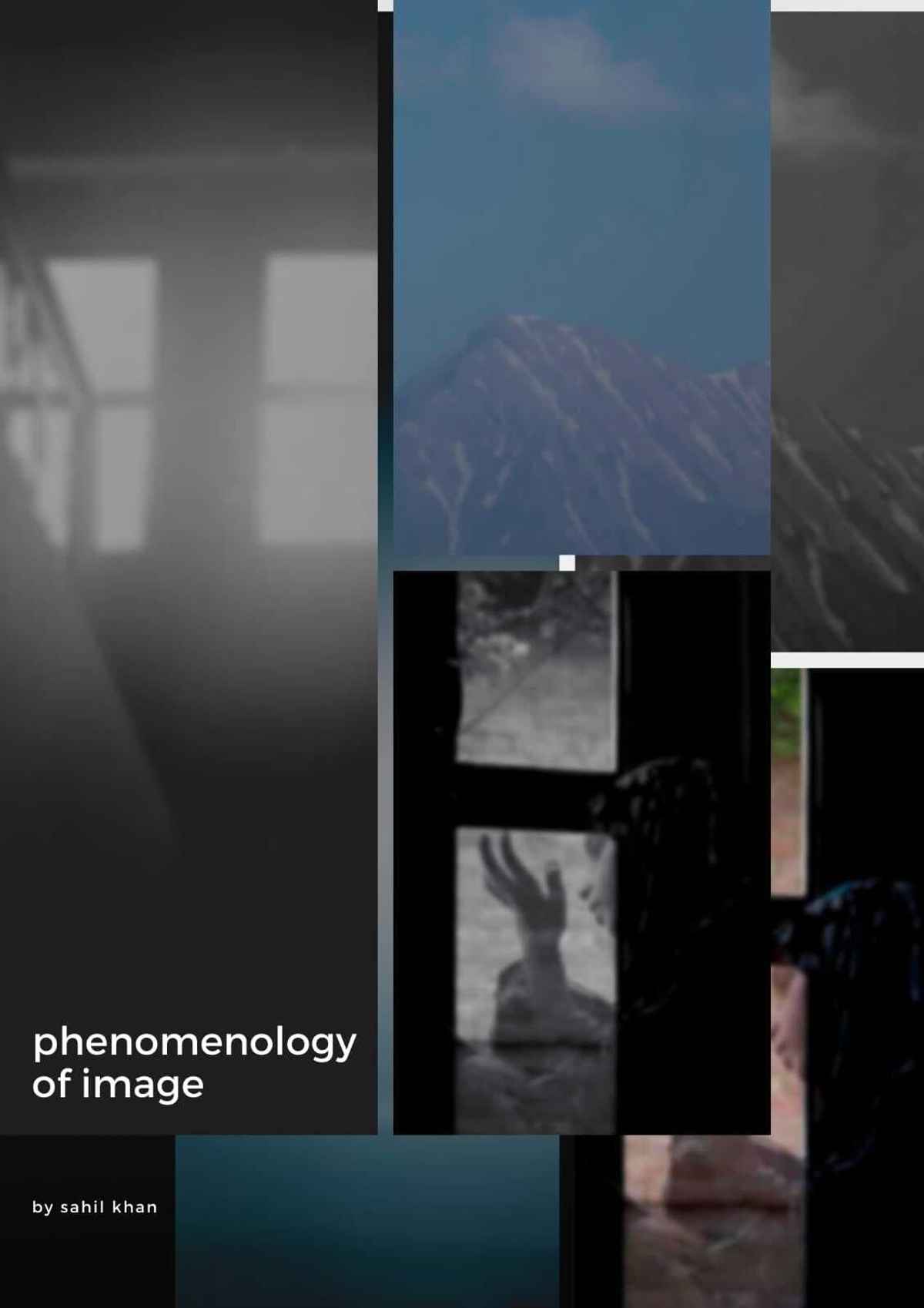The image is a detailed collage that likely serves as a book cover or an e-book cover, potentially also a website infographic. Titled "Phenomenology of Image" by Sahil Khan, the cover includes a composite of six distinct fragments, blending black, white, and blue tones. In the lower left corner, the title and author's name are prominently displayed. Among the images, there is a black-and-white faded photograph of a window, the interior of an old house with windows and a staircase, and a blurred portrayal of someone sitting contemplatively with their elbows resting on a table. Additionally, there's a duplicate image of the same person gazing out of a window, one in black and white and the other in color. The top right corner of the cover showcases a mountainscape with some snowpack, partially in gray with the peak set against a clear blue sky. These elements, overlaid and filtered together, create a cohesive yet fragmented visual narrative, emphasizing varied perspectives and contemplative moods.